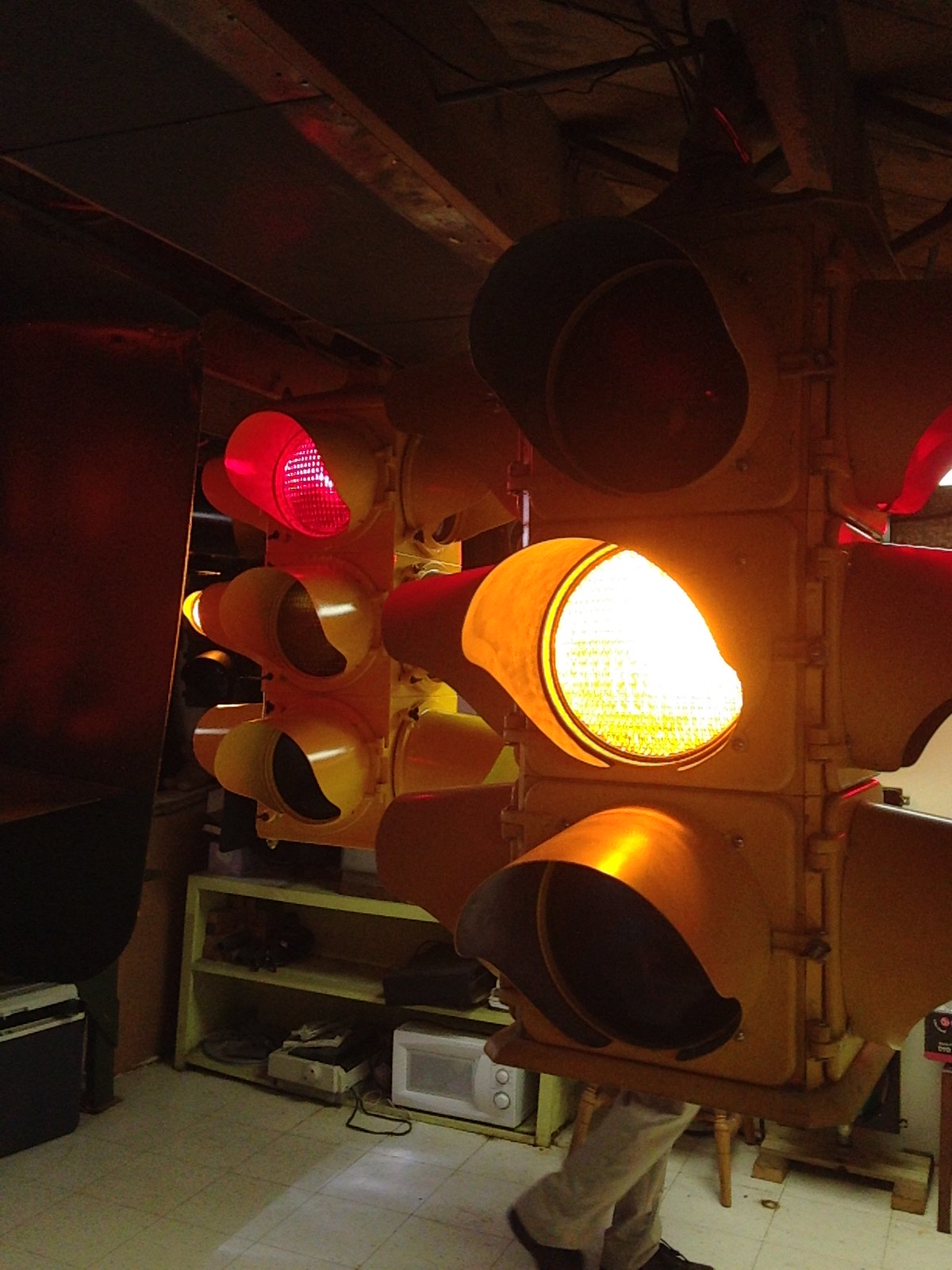The image depicts an unusual indoor setup featuring two traffic lights suspended from the rafters, akin to a basement environment rather than a street intersection. The traffic light in the background glows red, while the one in the foreground emits a white or yellow light. These lights provide stark illumination in an otherwise dimly lit room. A shelf laden with various appliances is situated behind the traffic lights, adding to the eclectic nature of the scene. The white tile flooring is visible, along with a pair of legs clad in beige slacks and black shoes. This striking scene, primarily defined by the red and yellow lights, casts dramatic shadows and highlights the distinct lack of illumination beyond the lights themselves, rendering the backdrop into obscurity.